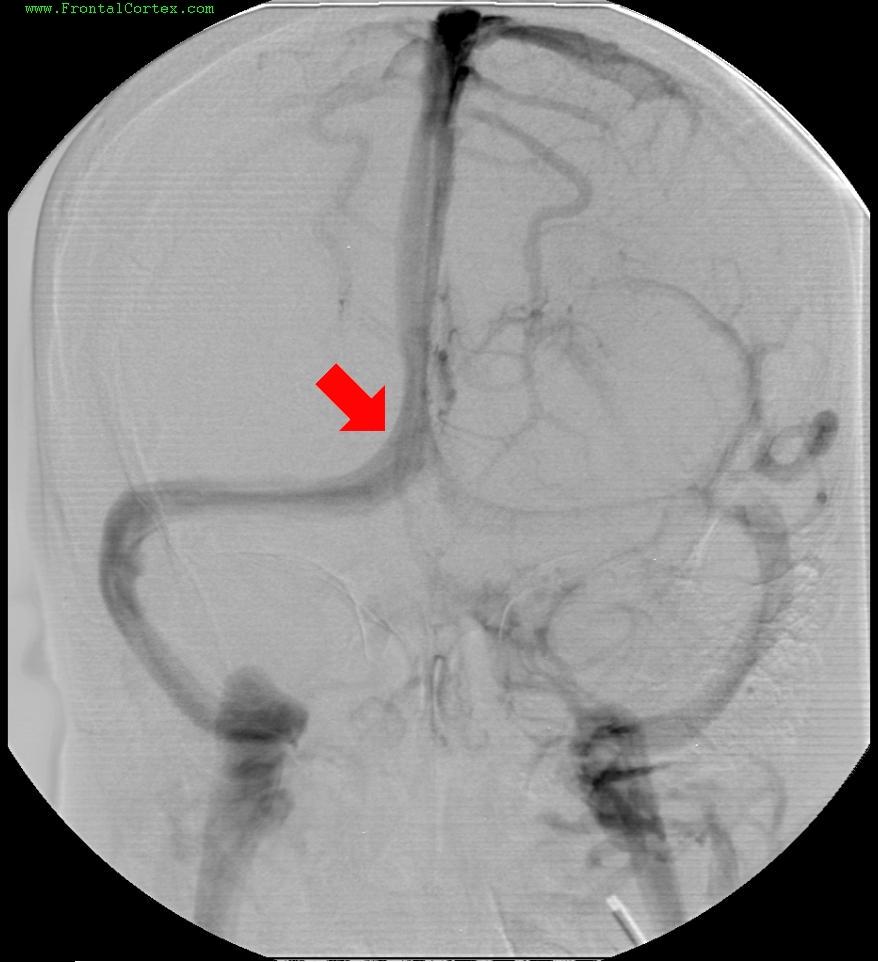This black and white microscopic image depicts a partially visible circular slide against a black background. Dominating the center is a series of wavy, organic lines, resembling blood vessels, capillaries, or plant roots. These lines run vertically down the image before branching out and curving back towards the center. A prominent red arrow is positioned at the focal point where the main line branches into two sections. The top left corner of the image features the green text "www.frontalcortex.com". The circular object appears cut off at the top, bottom, left, and right, but enough is visible to infer its round shape. The upper area of the image transitions to a darker shade, which continues towards the bottom left and right, where the branching structures also migrate into deeper tones before disappearing off the frame.